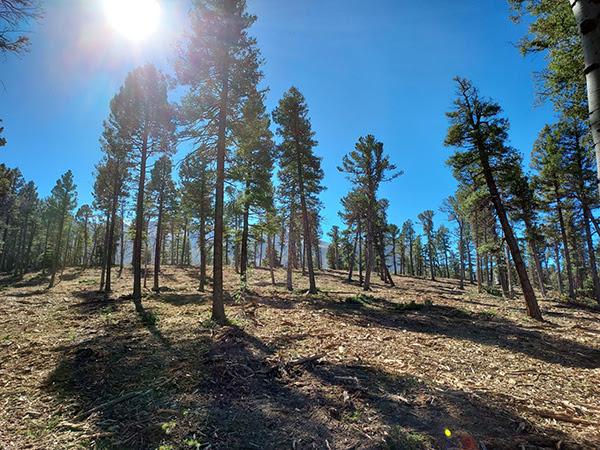The color photo captures a serene forested landscape bathed in bright, clear daylight. The sky, an unblemished expanse of blue, hosts the sun in its upper left corner, casting a luminous glow across the scene. The sparsely wooded area features an assortment of tall, young evergreen trees, likely fir or pine, with their foliage starting mid-trunk and tapering into pointed tops. These trees are thin and spaced out, suggesting that the forest may have been thinned over time, although denser tree lines can be seen in the background. A notable tree on the right leans slightly to the left, adding character to the composition. The ground, a mix of dirt and mulch, is strewn with sticks and devoid of grass, enhancing the natural, untouched feel of the setting. In the distance, partially concealed by the trees and the camera angle, the faint outlines of mountains rise, imparting a sense of depth and tranquility to the image. The sunlit scene, with its long shadows cast towards the viewer, radiates a calm and peaceful atmosphere.